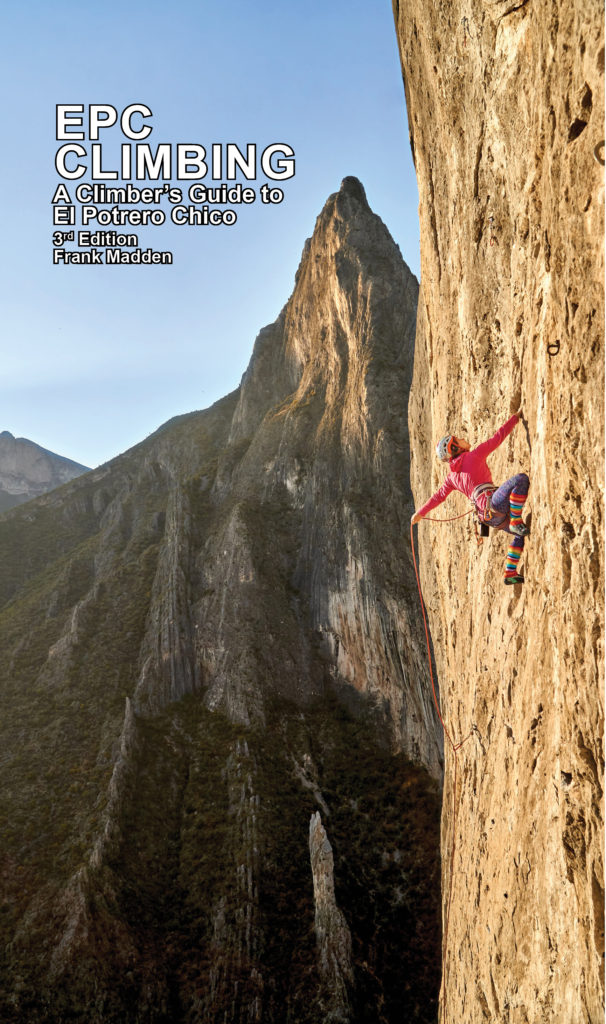The promotional image for "EPC Climbing: A Climber's Guide to El Potrero Chico, 3rd Edition" by Frank Madden features a stunning, realistic portrayal of a rugged mountain landscape under a clear, blue daytime sky. Dominating the scene is a woman climber in a pink sweater, scaling an imposing, flat beige cliff face adorned with small divots and rocky protrusions. She wears vibrant, knee-high striped socks in yellow, green, red, and orange, leopard-print purple leggings, and a gray and orange helmet, while her red hair flows behind her. Her right hand clutches the mountain surface as she leans back, her left arm trailing behind her. High above the ground, with no ground visible below her, she exemplifies the thrill and challenge of rock climbing. To her left, the background features towering, jagged mountain peaks, their upper sections brown and lower sections covered in green moss and grass. Overlapping this scenic backdrop, in the top left corner, is the promotional text: "EPC Climbing" in bold white capital letters outlined in black, followed by "A Climber's Guide to El Potrero Chico" in smaller white text, and "3rd Edition, Frank Madden" in even finer print.